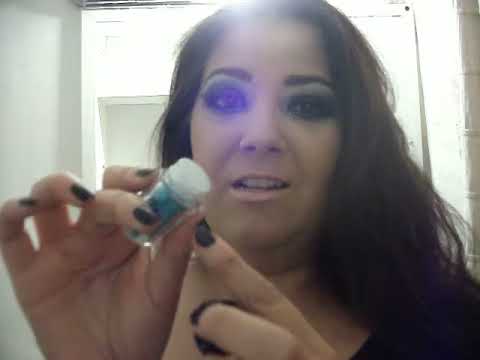This image appears to be a grainy, webcam screenshot featuring a middle-aged, fair-skinned woman with long, wavy dark brown hair and heavily applied eye makeup, including bluish eyeliner, dark eyeshadow, and thick eyelashes. She is dressed in a black shirt and has pale pink lipstick on her lips. The woman is in an indoor setting, likely a room with white or light gray walls, and there's a bright light source behind her, possibly a door or a back cabinet. 

In the immediate foreground, she holds a small, clear glass bottle with a white plastic stopper and blue substance inside, possibly a cosmetic product, in her right hand. Her black-polished nails are clearly visible, and her left index finger points to the bottle. She has her mouth open as if she is talking. Behind her, some shadows and what appears to be a brick wall can be seen to the right.